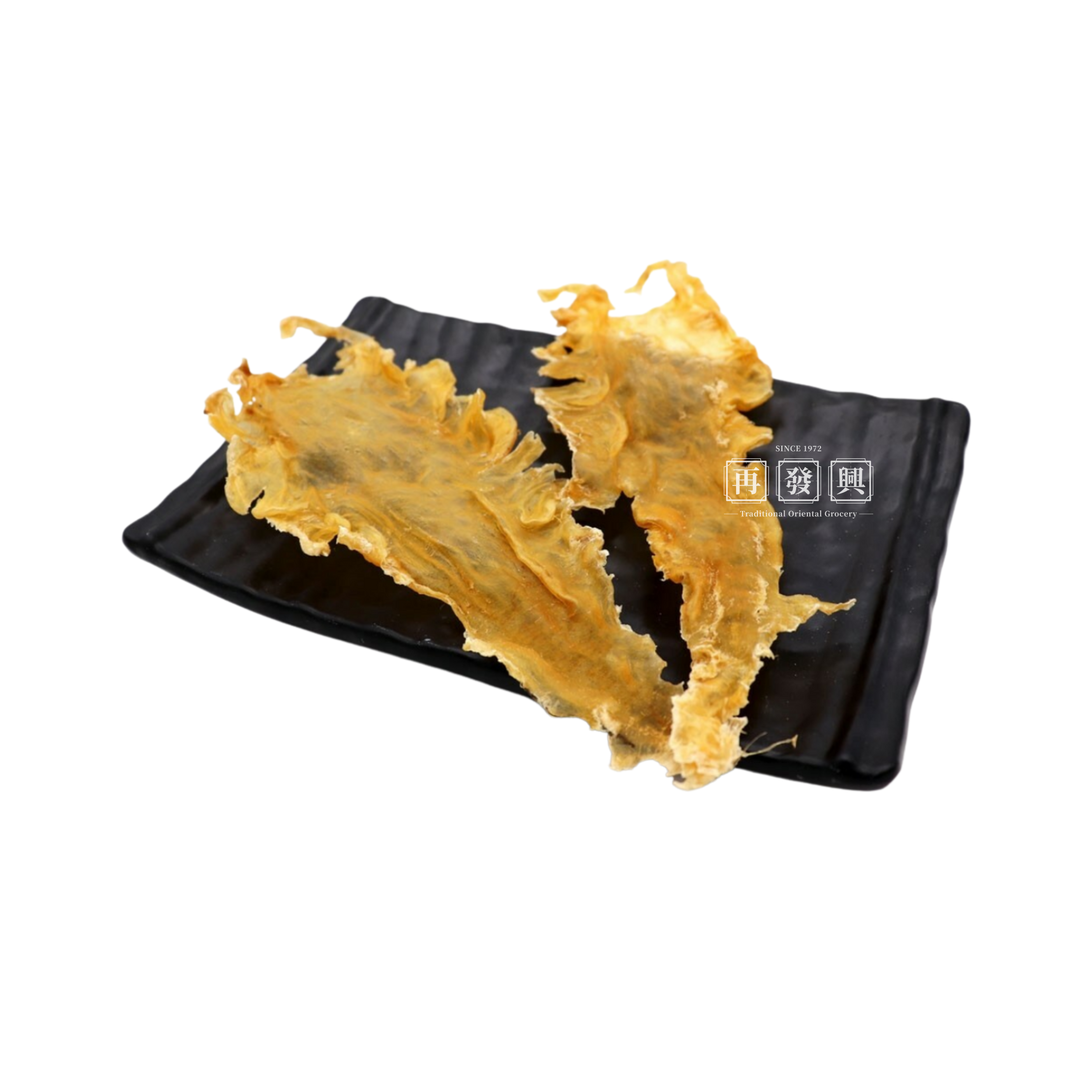In the image, a black mat, possibly made of plastic or cloth, is positioned against a stark white background and rotated slightly clockwise. Resting on the mat are two pieces of dried, brittle, yellowish-brown material that resembles fried chicken skin or some kind of dried meat. These pieces are irregularly shaped with zig-zaggy edges, suggesting a rough and dried texture. The mat itself has subtle lines running across it, adding some texture to its surface. Prominently displayed in white text over the image are the words "since 1972," followed by three squares containing Chinese characters, and underneath that, "traditional oriental grocery." This suggests that the dried pieces might be a product sold at this grocery store.